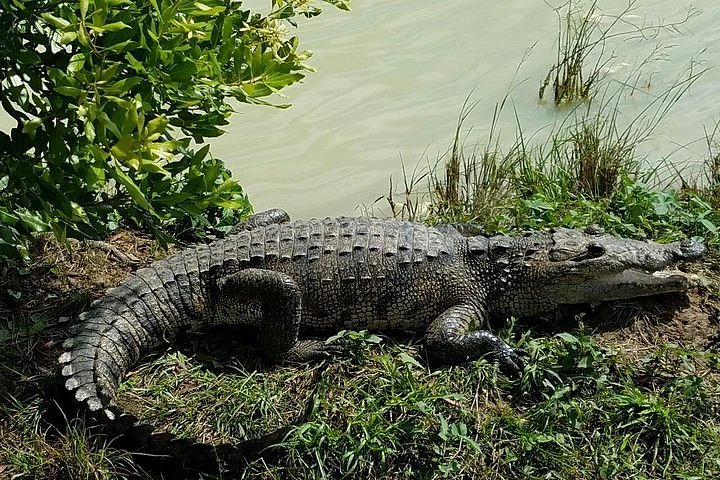An alligator basks in the sun, lying on a patch of short grass and weeds by a pond. His snout is distinctly rounded, differentiating him from a crocodile. His tail curls inward toward his body, and his slightly open mouth suggests he's trying to cool off on a warm day. The alligator appears aware of the photographer's presence. Behind him, a laurel tree offers a lush backdrop. The brown earth transitions into the nearby pond, which is bordered by tall sawgrass and reeds that continue into the water. This scene captures the tranquility and natural habitat of the alligator as it enjoys the sunny weather.